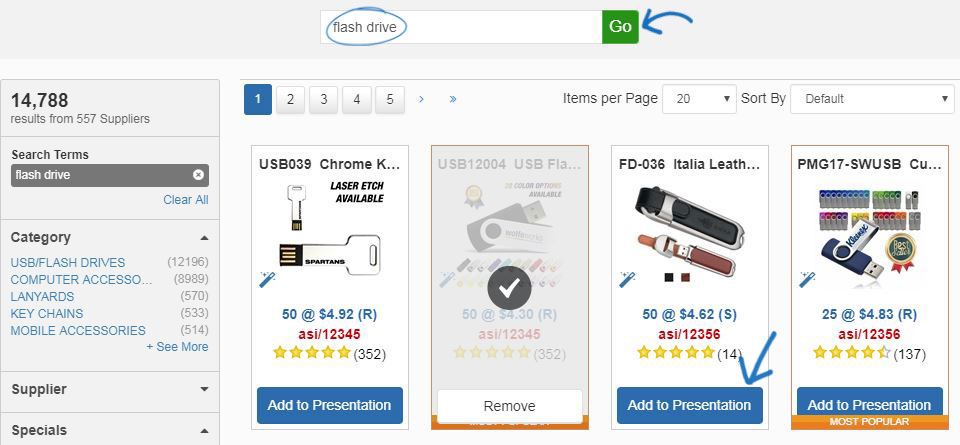The image displays a web page focused on the search results for "flash drive". At the top, the term "flash drive" is entered into the search box, which is circled in blue, emphasizing its importance. There is a green "Go" button next to the search box, with a blue arrow pointing towards it, indicating that the user should click this button.

On the left-hand side, there is a search results summary indicating "14,788 results from 557 suppliers". Below this, under "Search Terms", the phrase "flash drive" is displayed in a gray text box. There is also a blue "Clear All" button to reset the search.

Various categories are listed on the side, including USB Flash Drives, Computer Accessories, Lanyards, Keychains, Mobile Accessories, Supplier, and Specials, allowing the user to filter their search further.

The top section of the search results showcases four items with images. The first item resembles a key and a wrench. The second item, labeled "Italian Leather", includes two objects: one resembling a black flashlight and the other a smaller USB drive. The third item features a USB drive image with a tag, displaying text "25 at 483" and 137 reviews. A blue arrow directs attention to a button labeled "Add to Presentation", suggesting user interaction with this feature.

The overall page layout includes a white background with some gray boxes, typical of an online shopping website. The presented elements aim to guide the user through the search and selection process effectively.